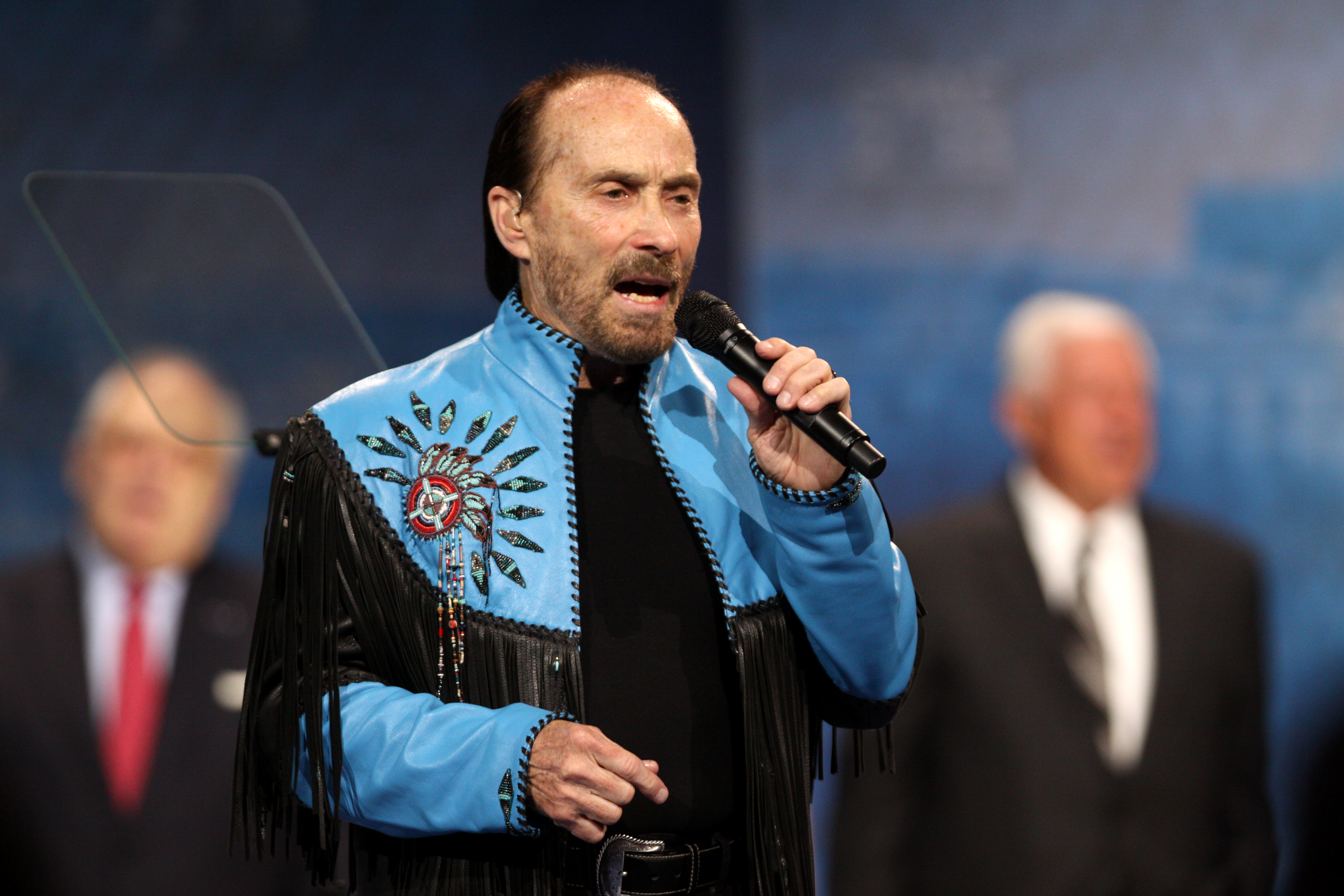In this image, a man stands at the center holding a microphone in his left hand. He appears to be in the midst of speaking, with his mouth open and his right hand bent at the elbow, pointing to the right. The man is balding, sporting dark hair on the back of his head, along with a beard and mustache. He is dressed in a distinctive fringed jacket, turquoise at the top with an Indian headdress design on the chest panel. The rest of the jacket is adorned with long black fringe. Underneath, he wears a black shirt and a black belt is partially visible. The setting appears to be an indoor event, possibly political, taking place during the day. The background, though slightly blurry, reveals some kind of signage or poster, and a few individuals in suits. The color palette of the scene includes shades of black, light blue, red, tan, gray, and silver, contributing to an overall formal and possibly significant atmosphere.